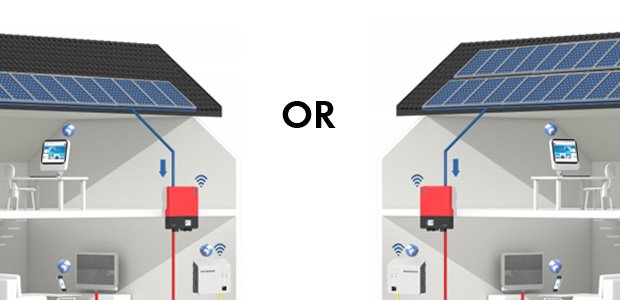The image depicts a mirrored, split-section illustration of a two-story house, showcasing the interior and exterior from two perspectives. Each side highlights the connectivity and energy flow within the house. On the left side of the image, the house has a single row of solar panels on the roof. A blue line with an arrow leads from these solar panels down to a red and black box featuring a blue Wi-Fi signal icon. From this box, a red line extends down to another white box with gray sides, which is marked with a drawing of the Earth and a Wi-Fi signal, symbolizing internet connectivity. This flow suggests the solar energy is powering connected devices inside, such as a computer, TV, and phone. The right side of the image mirrors this setup but features two rows of solar panels instead of one. The image is set against a white background, with the word "OR" prominently displayed in the middle in black text, suggesting a comparison between the setup with one row of solar panels versus two rows.